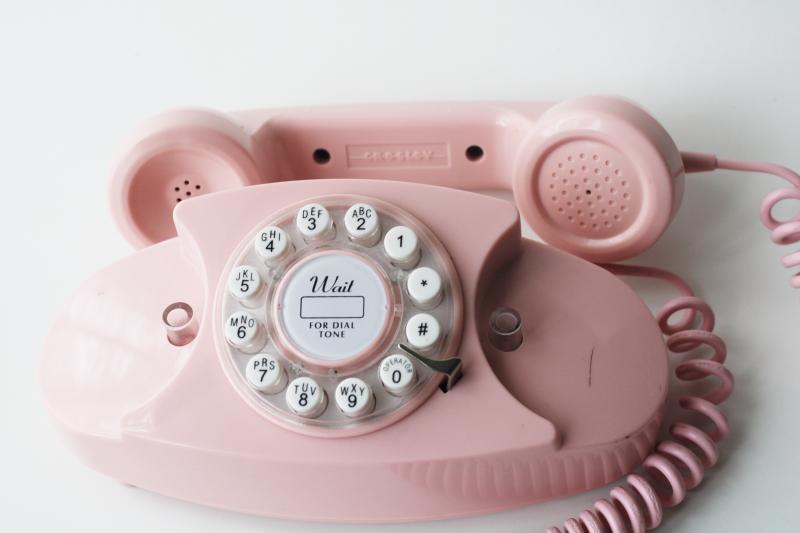The image showcases a vintage pink rotary phone placed on a table against a pure white background. The phone's base and handset are both pink, as is the coiled telephone cord. The rotary dial displays white circles with black text, specifying numbers from 1 to 9, along with the corresponding standard lettering (e.g., ABC for 2, DEF for 3), while the number zero is labeled as "operator." At the center of the rotary dial, the instructions "wait for dial tone" are printed in black around a small pink circle. The handset is detached from the base, resting next to it, with the earpieces visible. The base of the phone also features two clear cylindrical pieces where the receiver would typically rest, connecting to holes in the receiver. There's also a silver pin present to stop the rotary dial when dialed. The entire scene is lit with natural light, accentuating the pristine and delicate appearance of the pink phone against the stark white background.